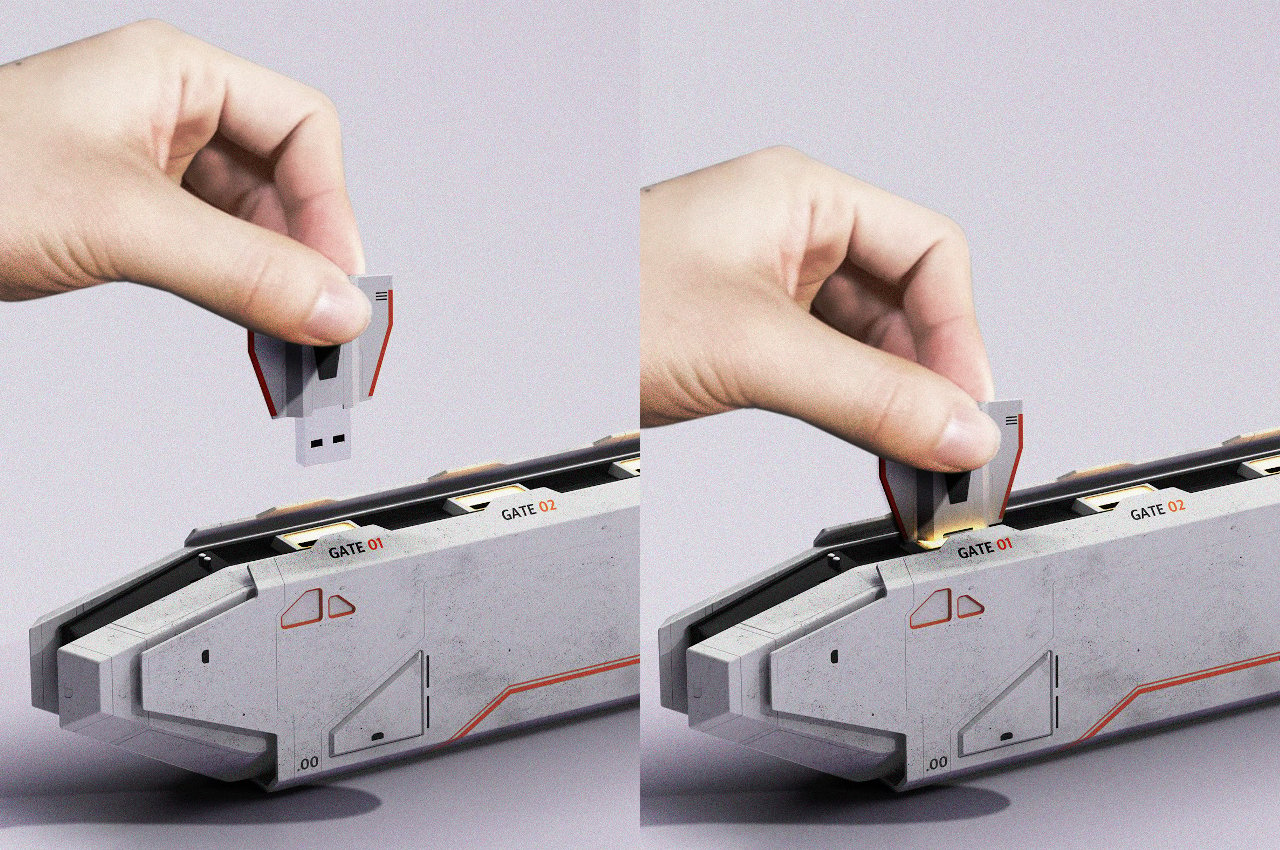The photo comprises two adjacent images, likely from an instruction manual, illustrating the process of inserting an object. On the left, there is a light gray metallic strip with some red striping, resembling a toy spaceship, lying horizontally on a table. The strip features three visible ports, with the labels "gate 1" and "gate 2" in black text, and the numbers in red text. A hand reaching in from the left side is holding a USB-like chip with wing-like extensions and orange stripes, positioning it above the "gate 1" port. In the right image, the hand has moved to insert the chip into the "gate 1" port, illuminating a light exactly where the chip is now connected, while "gate 2" remains unoccupied. The gray background and nearly identical composition of the images emphasize the action sequence of the chip being plugged in.